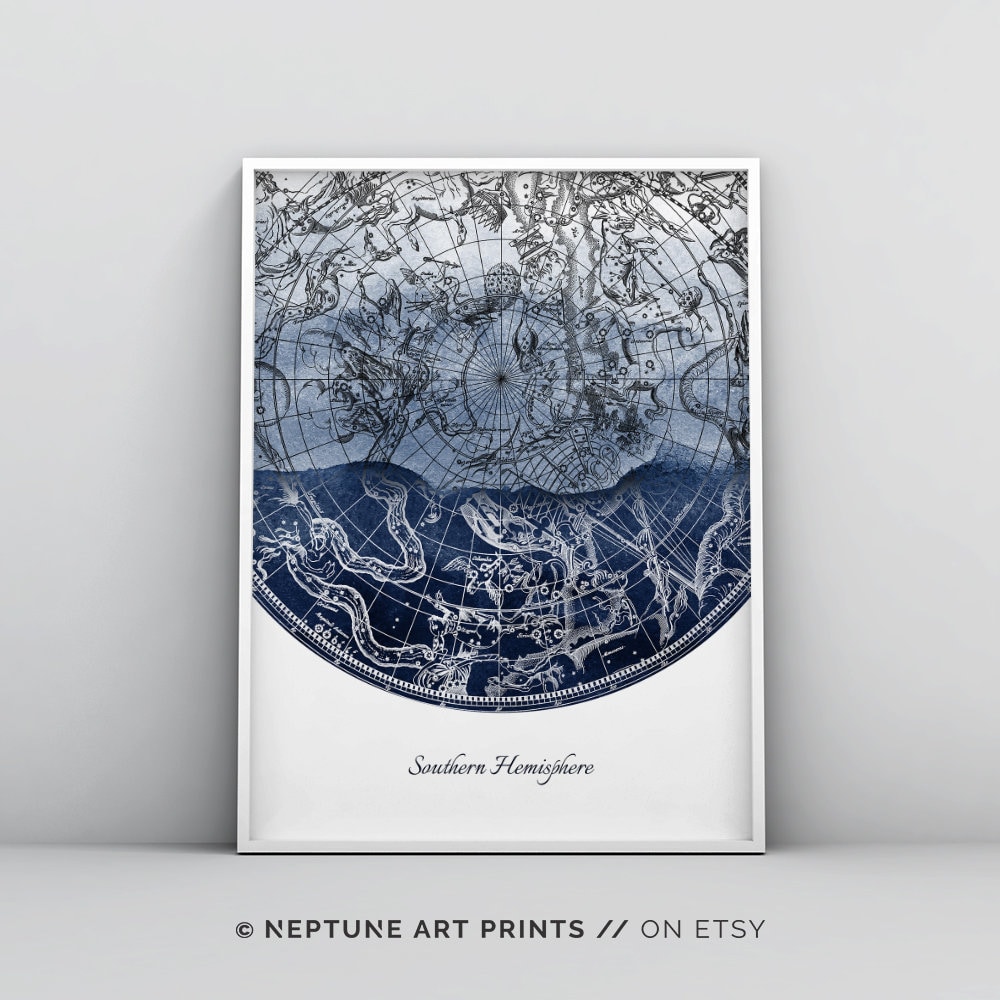The photograph depicts a framed artwork leaning against a gray and blue backdrop. The narrow, white frame holds an intricate and detailed depiction of the Southern Hemisphere. Central to the piece is a globe-like circle with a grid of latitude and longitude lines converging at a focal point, creating a web-like pattern. The bottom of the circle is blue, transitioning to gray and white towards the top. The sphere is adorned with a myriad of random shapes, scribbles, and ambiguous sketches, some of which resemble animals like serpents, camels, and whales, though many are indiscernible.

At the bottom of the image, within the frame, blue cursive text against a white background reads "Southern Hemisphere." Below the frame, overlaid on the photograph, black text states, "Copyright Neptune Art Prints // on Etsy." The combination of grid lines, diverse shapes, and layered text creates a visually compelling and enigmatic piece that is both detailed and abstract.